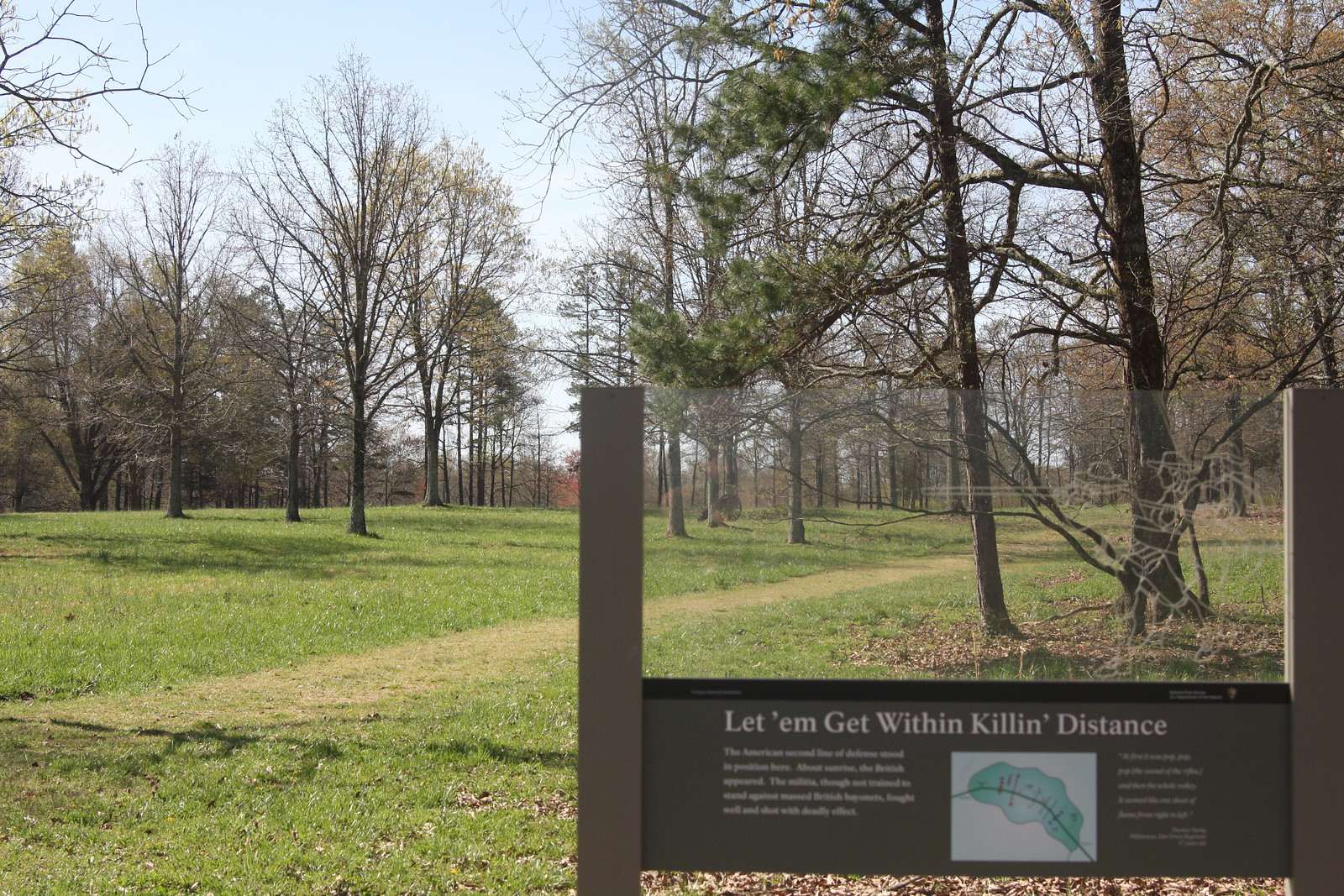The image depicts a serene park scene on what appears to be a clear fall or winter day. The grass is bright green but appears short, suggesting it hasn't grown much recently. Trees without leaves stand in the background, contributing to the sense of it being a quieter season, though the sky is a light blue, indicating good weather. Dominating the foreground is a signboard supported by two wooden posts with a glass panel in the middle. The glass section features etchings of 19th-century soldiers with long rifles, suggesting a historical context, possibly of a past war. Below the etchings, the prominent text reads "Let them get within killing distance" in Times New Roman font, with smaller, unreadable text beneath it. The sign also includes an image of a green leaf or possibly a map, although details are blurry. A paved pathway with bits of grass peeking through winds across the scene, contributing to the park’s peaceful and empty ambiance – an ideal spot for a tranquil walk.